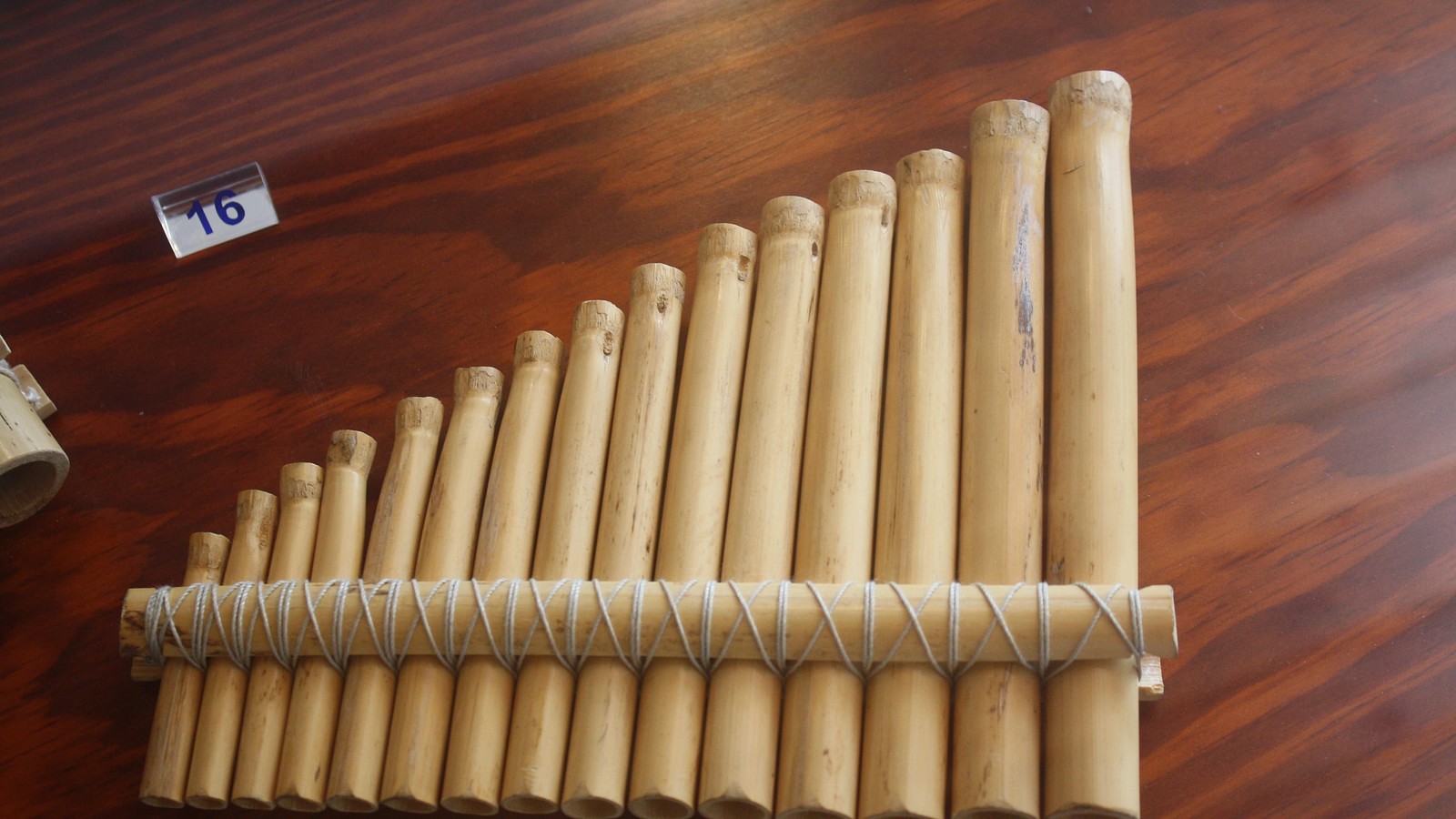This is a detailed color photograph of a primitive wooden musical instrument, likely a pan flute, displaying a collection of wooden sticks of varying lengths. The sticks are arranged side by side, increasing in height from left to right, and are bound together with white string on both ends. Additionally, a horizontal piece of wood is tied around the instrument for added stability. The instrument, made from light wood, is positioned on a dark brown wooden table with a rich pattern. At the top left corner of the image, there is a tag marked with the number 16. No people, animals, buildings, or motor vehicles are present in the image.